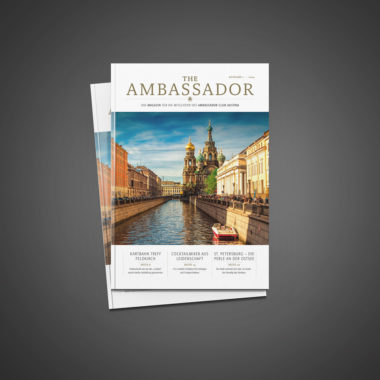The image depicts a book titled "The Ambassador" centered against a very dark gray, almost charcoal background, giving it a framed effect. The book appears to be thin and magazine-like, with a cover that prominently features a picturesque canal scene—likely Venice, Italy. The canal is flanked by old-fashioned buildings; notably, there's a tan building and a red boat on the right side. However, the architectural style suggests it could also be another city, perhaps in Russia or the Netherlands, as there's a domed building resembling a Russian cathedral off to the right. The title "The Ambassador" is written in gray text on a white strip across the top of the cover, which also has a white strip at the bottom containing blurred text that appears to be divided into three columns, most likely indicating the authors or book topics. The background book is almost entirely obscured, with only the one in front being clearly visible.